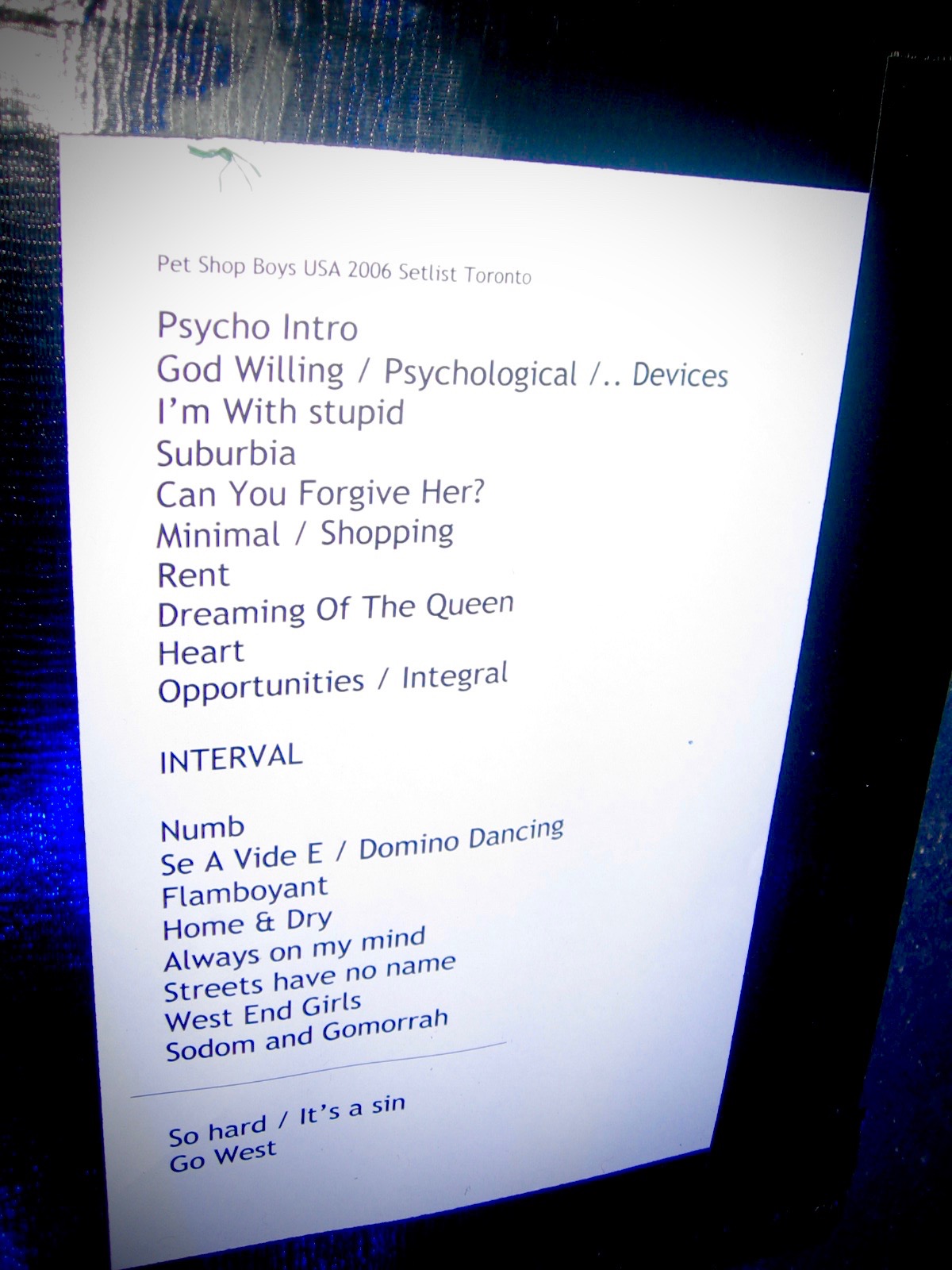The image depicts a printed setlist pinned to a wall, likely illuminated by a light source, causing the white paper to reflect brightly against a dark blue background. The text is aligned to the left in black font. At the top, it reads "Pet Shop Boys USA 2006 Setlist Toronto." Below this heading, the setlist begins with "Psycho Intro" followed by "God Willing," "Psychological," and "Devices." The list continues with songs: "I'm with Stupid," "Suburbia," "Can You Forgive Her," "Minimal," "Shopping," "Rent," "Dreaming of the Queen," "Heart," and "Opportunities" / "Integral." 

An interval divides the setlist. Post-interval, additional songs are listed: "Numb," "Say a VDE," "Domino Dancing," "Flamboyant," "Home and Dry," "Always on My Mind," "Streets Have No Name," "West End Girls," and "Sodom and Gomorrah." The setlist concludes with "So Hard" / "It's a Sin" and the final song "Go West."